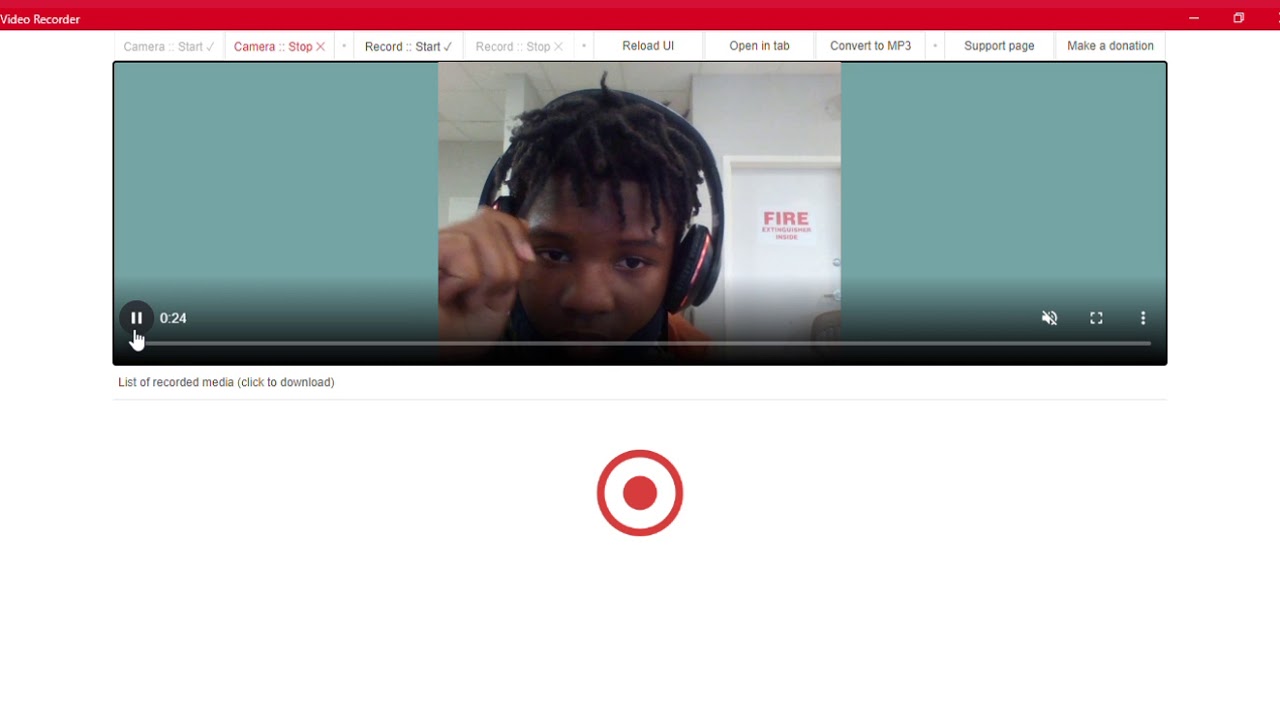This detailed screenshot captures the interface of a video recorder site. At the top of the interface, there are several buttons labeled "Camera," "Start," "Check," "Camera," "Stop," and an "X" in red. Below them, additional options are displayed, including "Record Start," "Record Stop X," "Reload UI," "Open in Tab," "Convert to MP3," "Support Page," and "Make a Donation." Notably, the top bar is highlighted in red.

A video player occupies the main section of the interface, with the mouse cursor hovering over the pause button at the 24-second mark. The video is muted, as indicated in the bottom right corner of the player, and it is not in full screen mode. Adjacent to the video player, a "sandwich" (menu) button is visible.

The video itself features an image of a boy in an orange shirt wearing headphones, with his hand partially obscuring the camera. In the background, a door is labeled with the text "Fire Extinguisher Inside."

Below the video player, a section titled "List of Recorded Media" provides an option to click and download media files. There is also a prominent red record button, represented by a filled-in red circle with a border.

The interface is set against a blue background, providing a visually distinct frame for each element.